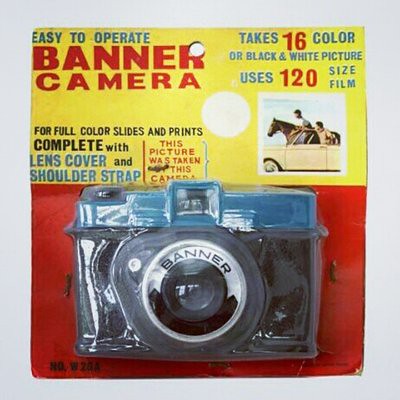This image features a vintage Banner camera prominently displayed in its original packaging. The black camera, set against a striking red background, is encased in a clear plastic see-through container. The camera's lens bears the brand name "BANNER" in bold letters. The packaging itself is square-shaped with a yellow top half that features red and blue printing, reading "BANNER CAMERA" and detailing its capabilities: "easy to operate," "takes 16 color or black and white pictures," and "uses 120 size film for full color slides and prints." Additional text indicates that the camera comes complete with a lens cover and shoulder strap. The product appears to be aimed for sale, captured in a photo with a gray backdrop. The overall setting suggests a vintage aesthetic, despite its toy-like appearance.